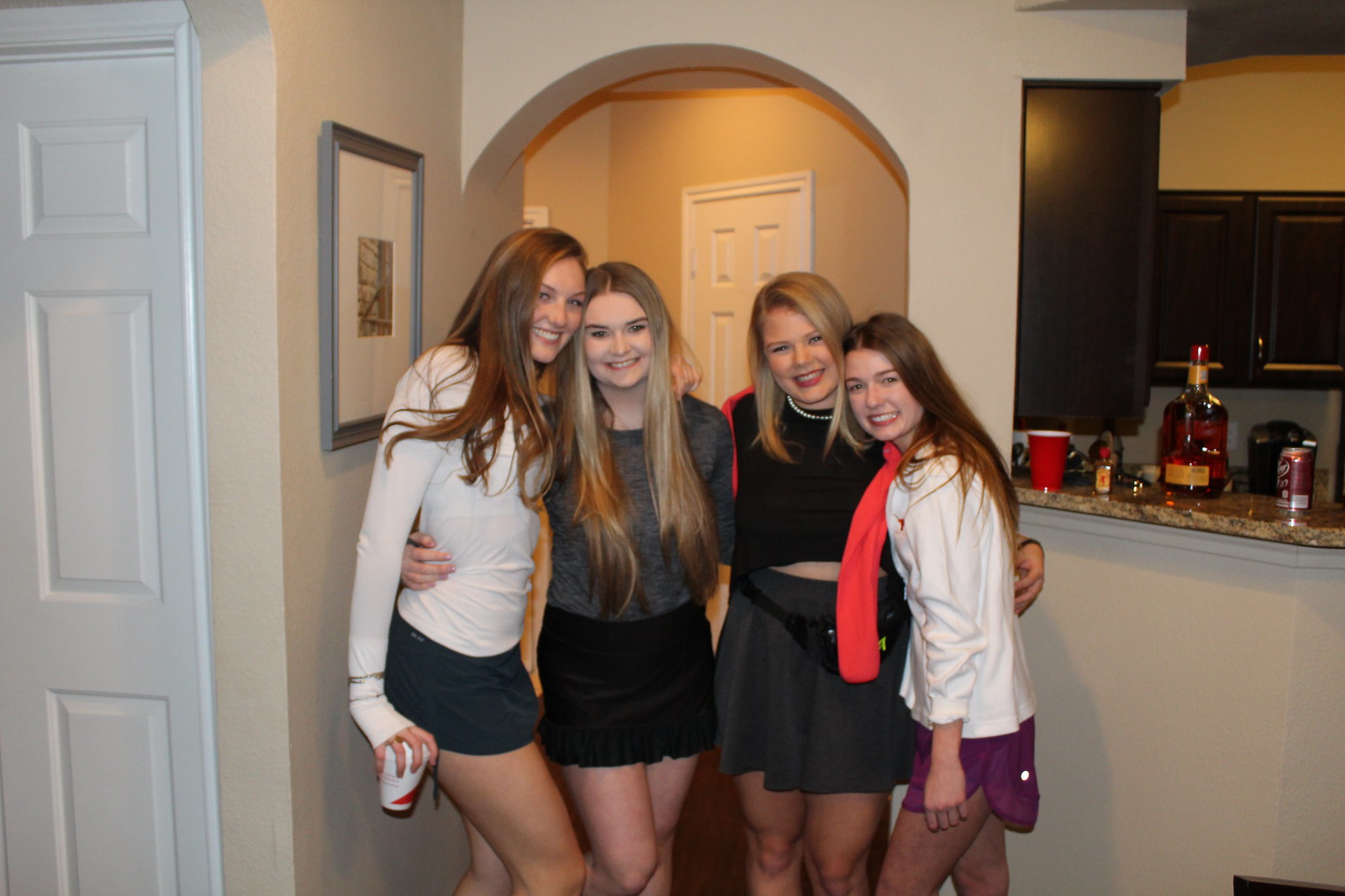In this detailed photograph, four young Caucasian women are standing together in front of an arched doorway, likely in a residential house or apartment. They are all posing and smiling for the camera, with their arms around each other. 

From left to right: The first woman has long brown hair and wears a white long-sleeve top paired with a black miniskirt, holding a cup in her left hand. Next to her stands a woman with waist-length blonde hair, clad in a gray shirt and black miniskirt. The third woman, sporting short blonde hair, is dressed in a black shirt and black miniskirt. The woman on the far right has brown hair and is wearing a white shirt with purple shorts.

To the right of the women is a kitchen bar area featuring dark cabinetry and white walls. On the beige-patterned granite countertop, various items are visible, including a large bottle of liquor, a red Solo cup, and what appears to be a can of soda. Additionally, there's a painting on the wall to the left of the doorway, enhancing the cozy and casual atmosphere of the scene.